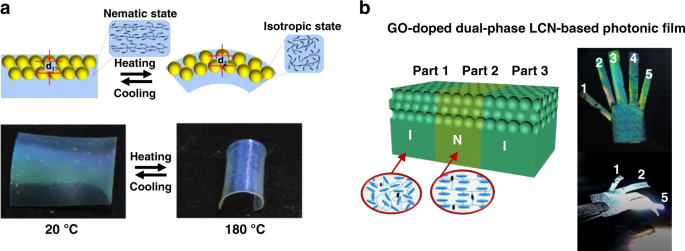The image is a detailed schematic advertisement for a product involving pneumatic and isotropic states of molecules, heating, cooling processes, and a go doped dual-phase LCN-based phototonic film. The left side features six images depicting different states of yellow circular molecules with annotations such as "pneumatic state" and "isotropic state," alongside arrows indicating heating and cooling directions, with temperature labels of 20°C and 180°C. There's also a blue box with yellow molecules marked with a "D" and a red cross, and another box showing squiggled lines representing different molecular states.

The right side of the advertisement emphasizes the go doped dual-phase LCN-based phototonic film, divided into parts one, two, and three. It includes images of green structures with blue components, labeled with "I," "N," and "I." Below this, there is a diagram of a glove with numbered fingers (1 to 5) and another hand diagram marked 1, 2, and 5, representing various stages or components of the phototonic film. The details in the schematic indicate specific molecular configurations and phases, crucial for the function of the phototonic film the advertisement aims to promote.